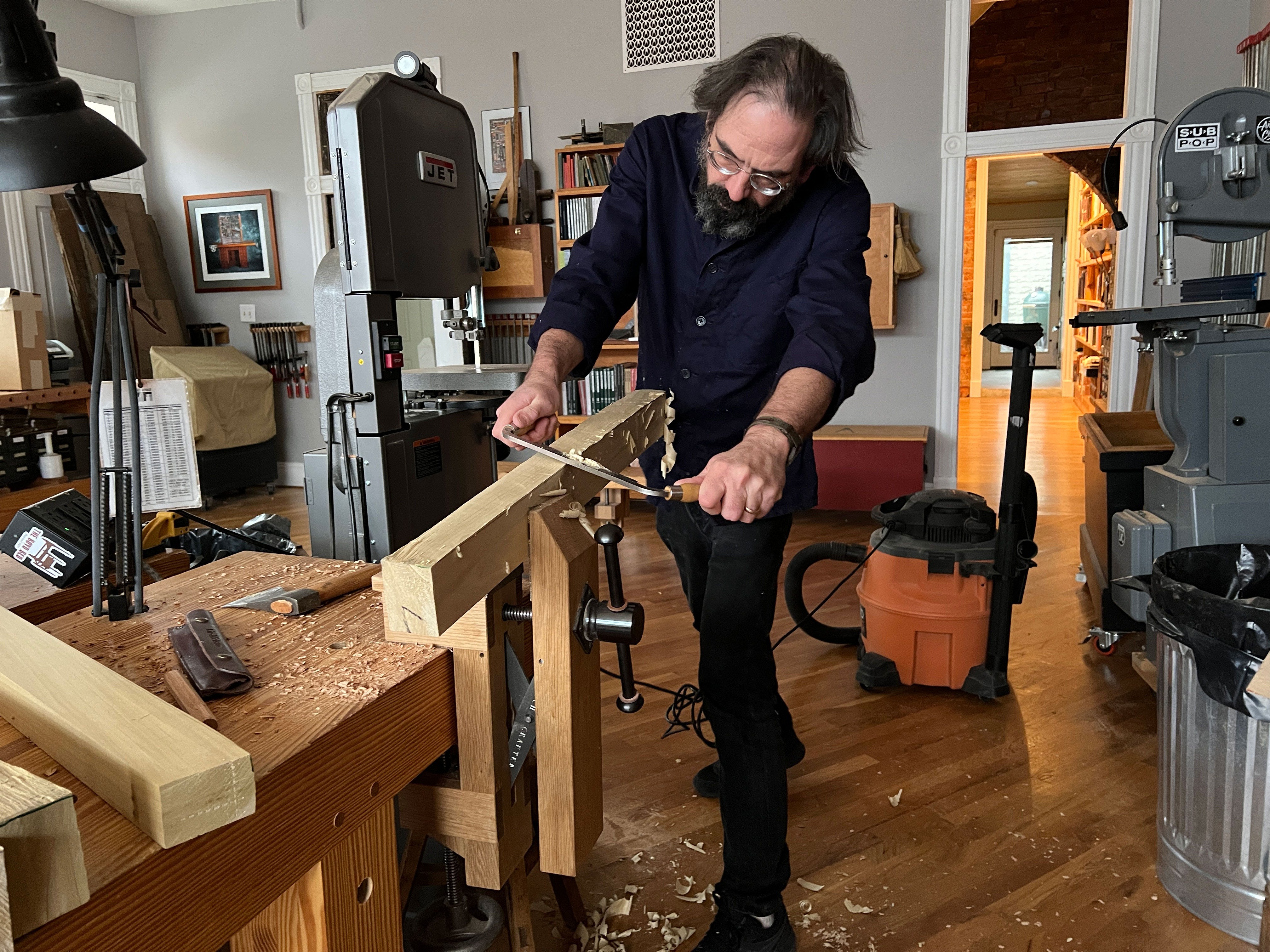This color photograph captures a middle-aged white man engaged in woodworking inside a room of his house. With long dark gray hair, a full black and gray beard, and round silver glasses, he is meticulously planing a board held in a wooden vice attached to a workbench. His workbench, cluttered with tools including a hatchet and a leather case, also holds several wooden planks, approximately two by two by three in size. Wearing black jeans and a black button-up shirt, the man is surrounded by various woodworking equipment, including a large gray drill press labeled "Jet". Also visible is an orange shop vac and an aluminum trash can with a black trash bag to his right. Behind him, bookshelves and framed pictures adorn the gray walls, indicating the room's dual purpose as a living space. The room features hardwood floors covered with wood shavings, underscoring his active project. A hallway is visible in the background leading to a back door, with daylight streaming in, further highlighting the domestic setting.